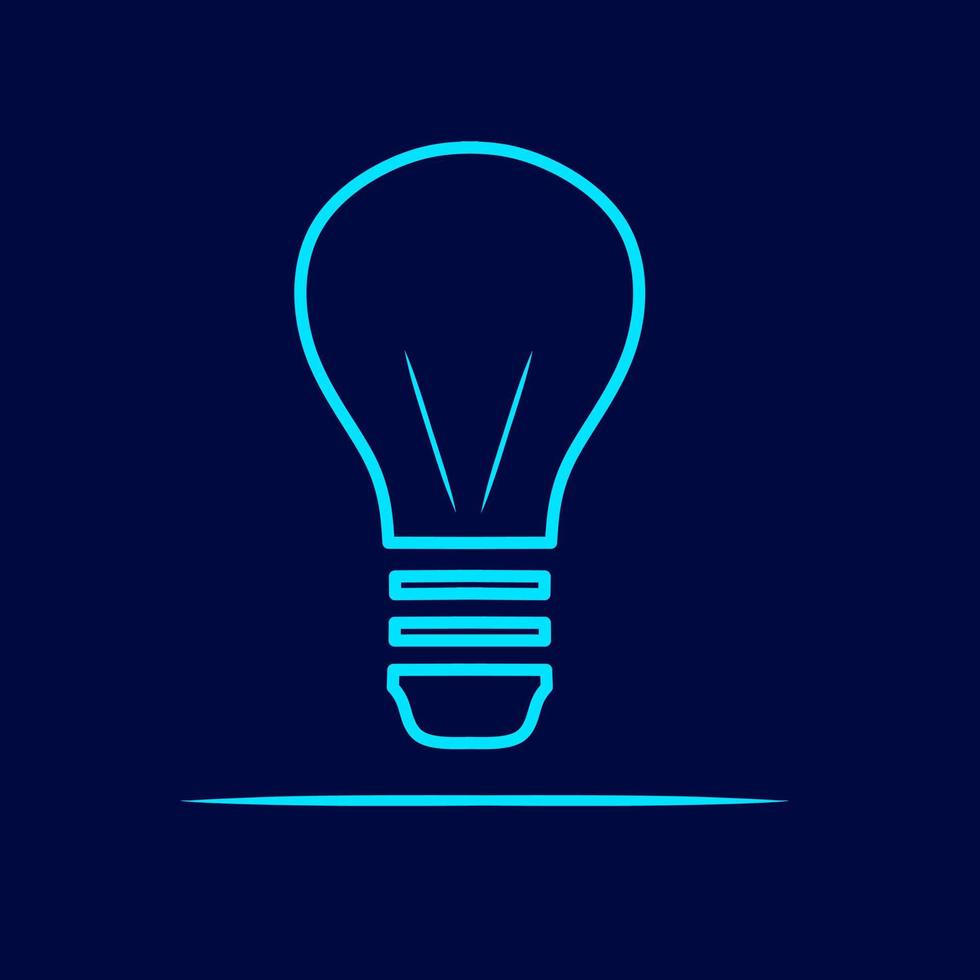This image features a detailed color illustration of a light bulb rendered in a light teal blue on a dark blue square background. The depiction of the light bulb is segmented into four distinct parts. The topmost section of the bulb displays two V-shaped lines that resemble filaments; these lines are placed within the lightbulb's outline. Additionally, two rectangular shapes, which float independently, are positioned between the V-shaped lines and the bottom section. This lower section mimics the screw part where the bulb would be inserted into a socket, represented by two parallel horizontal lines akin to an equal sign. Beneath the bulb outline, there is a solitary tapered line running horizontally across the image, accentuating the separation between the bulb and the base area. The overall rendering is characterized by its geometric style, with sharp, well-defined lines and shapes contributing to an organized and visually cohesive representation of the light bulb.